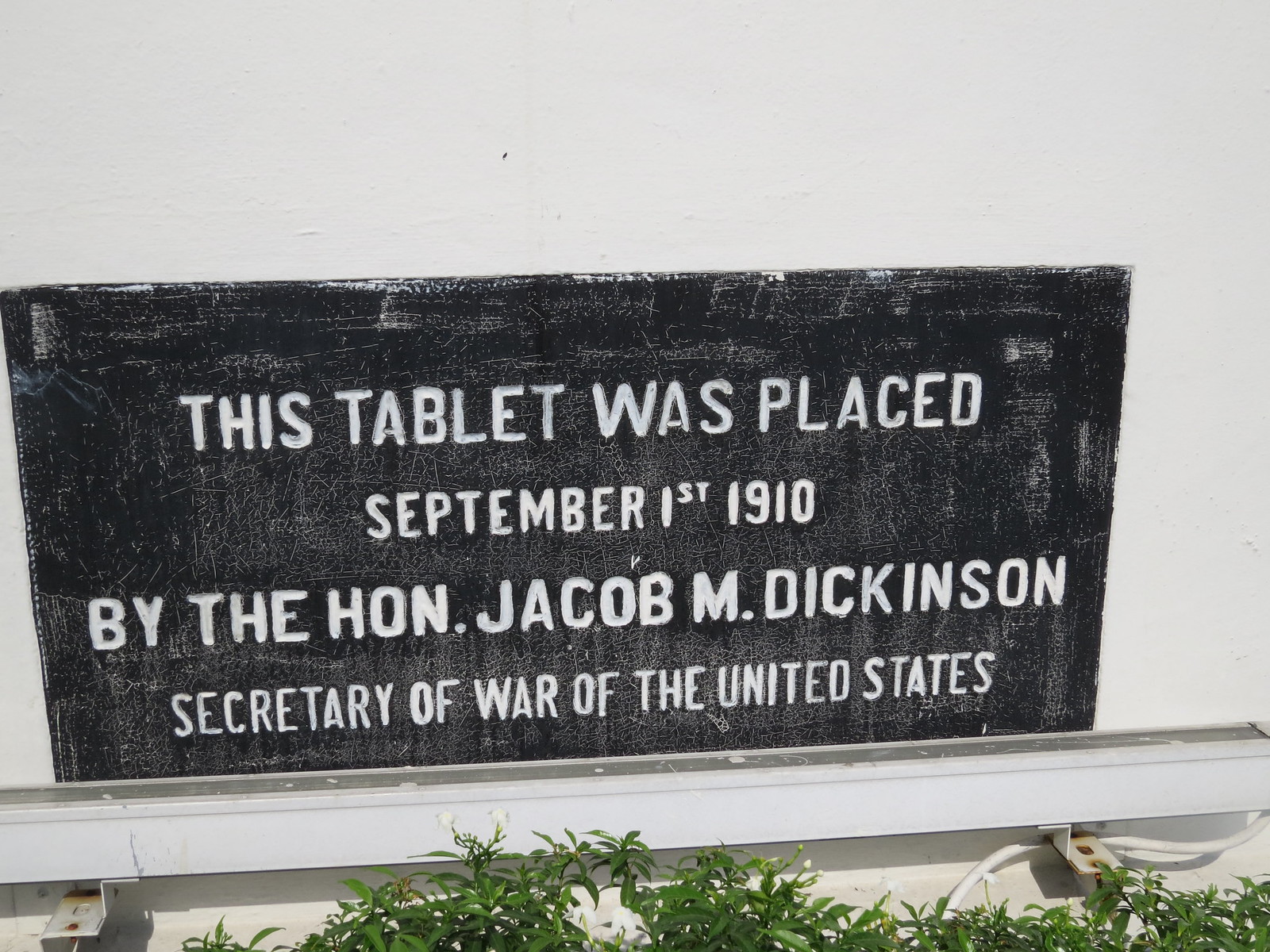The image depicts an older black stone plaque mounted on a white wall, prominently positioned on a ledge with green vegetation, including branches, shrubs, and grass, growing underneath it. The plaque, which takes up most of the frame, features an inscription in white uppercase letters: "This tablet was placed September 1st, 1910 by the Honorable Jacob M. Dickinson, Secretary of War of the United States." The text appears to be filled in with white chalk for clarity. Notably, there are two small bars protruding from the left and right sides beneath the placard, and a visible wire or cable runs adjacent to the right-side bar.